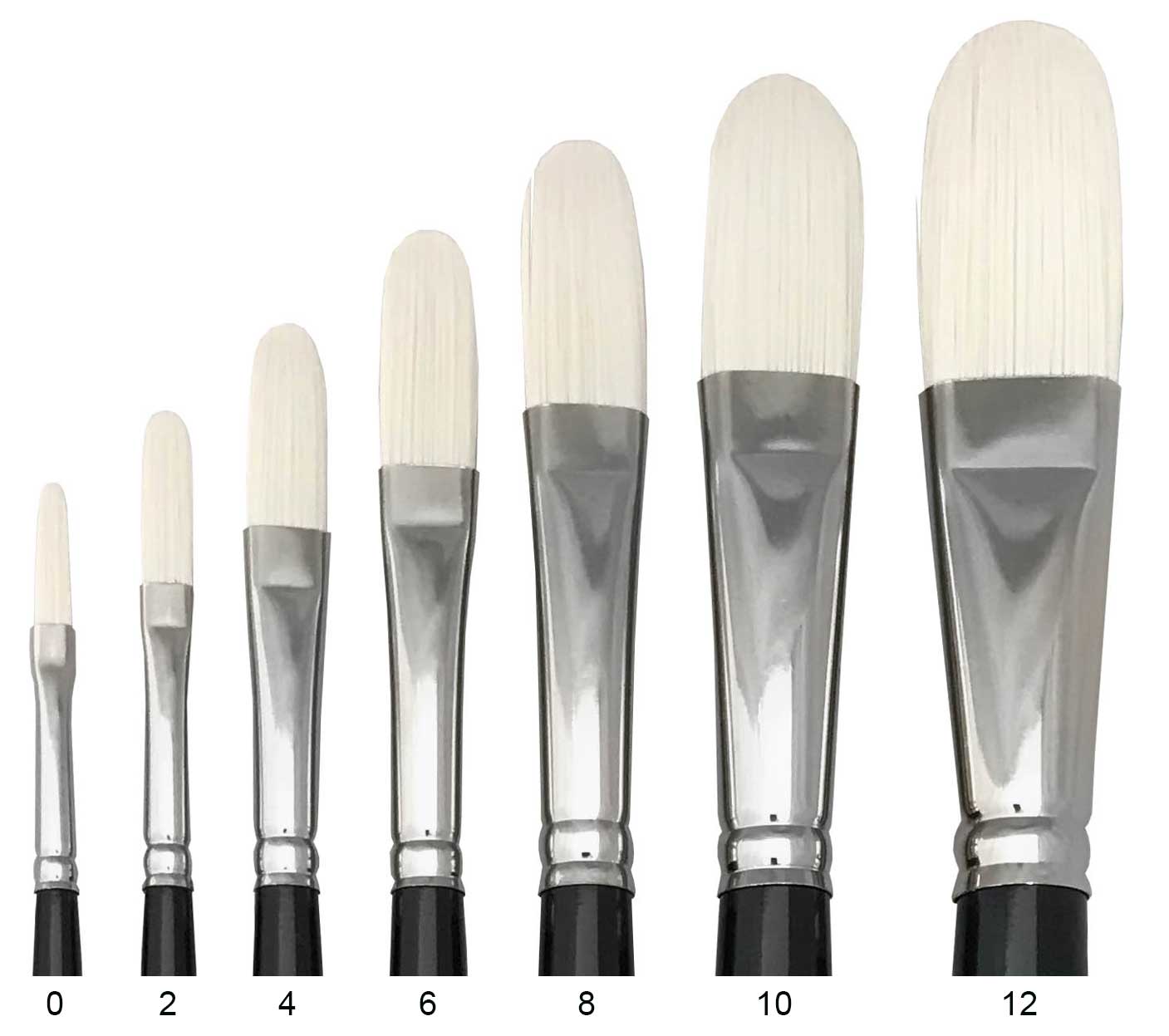In this image, seven paintbrushes are carefully arranged side by side from left to right against a solid white background. The paintbrushes vary in size, with the smallest on the far left and the largest on the far right. Each brush features a black handle, a silver ferrule, and light cream bristles. The brushes are numbered beneath each handle in black ink, reading 0, 2, 4, 6, 8, 10, and 12 consecutively from left to right. As the numbers increase, both the length and width of the brushes progressively grow, with the bristles becoming larger and taller. This orderly display emphasizes the gradual transformation in size and thickness of the paintbrushes.